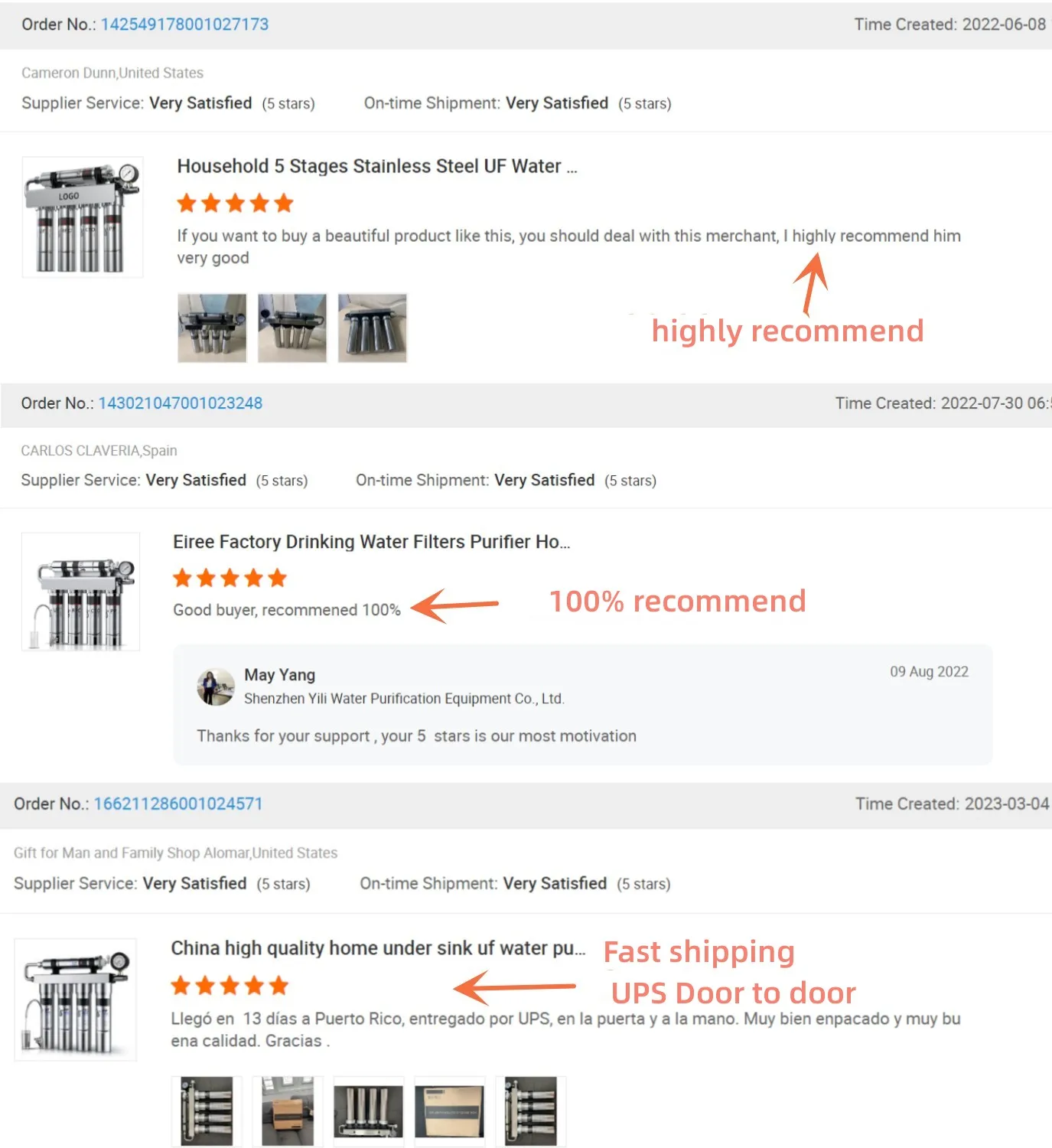The image displays a detailed review layout for three products, each marked by a light gray bar running horizontally across the top.

**Top Section:**
- The top left corner contains the text "Order Number" highlighted in blue.
- On the right side of the gray bar, the "Time Created" is indicated.
- Below the order number, the first product is reviewed as follows:
  - **Supplier Service:** Rated "Very Satisfied" with five stars.
  - **On Time Shipment:** Also rated "Very Satisfied" with five stars.
  - **Review:** Accompanied by three images of the product, the review states "Highly Recommend" with an orange upward-pointing arrow on the right.

**Middle Section:**
- For the second product, there is another five-star review with text stating "100% Recommend."
  - An orange arrow pointing to the left is next to this statement.
  - The review is attributed to May Yang.

**Bottom Section:**
- The bottom product is labeled "China High Quality Home Under Sink of Water PU..."
  - It has received a five-star review in red text: "Fast Shipping UPS Door to Door."
  - An orange arrow pointing left is situated next to this text.
  - Five images of this product are displayed below the review.

All the content is set against a clean white background, enhancing the readability and visual organization of the information.